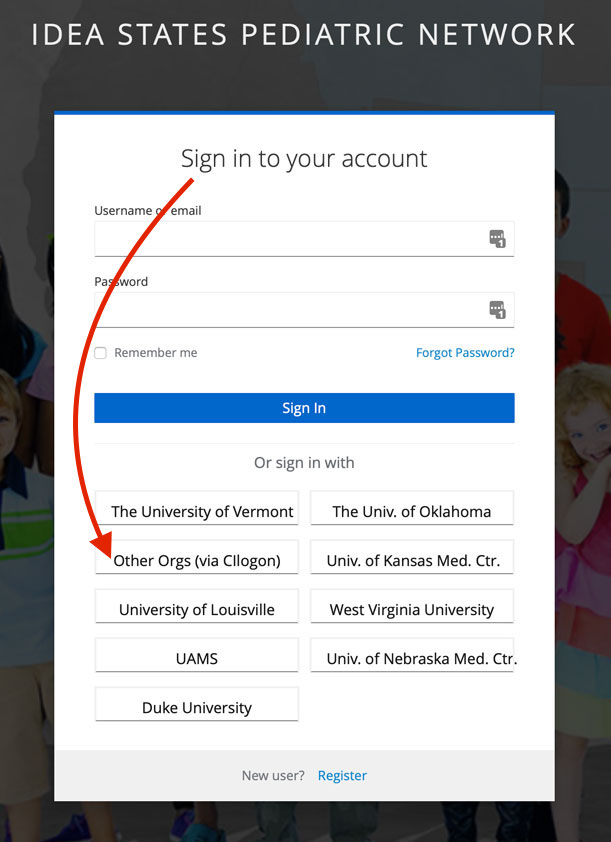The web page depicted is the sign-in page for the IDEA States Pediatric Network. The page is dominated by a prominent vertical rectangle featuring images of children and families, suggestive of pediatric care and support. Superimposed on this background is a vertical white box.

At the top of the white box, in bold black text, it states "Sign in to your account." Directly below this header, there are two horizontal input fields; the first is designated for the username or email, and the second for the password. Options to stay signed in are available via a checkbox labeled "Remember me." Adjacent to this, in blue text, is the option "Forgot password?"

Beneath the password field is a bright blue "Sign In" button with white text. Lower on the page, still within the white box, there is a section suggesting alternative sign-in methods with the prompt "Or sign in with." This section presents two vertical columns of buttons, each representing a different institution or service provider: University of Vermont, other organizations via Silicon, University of Louisville, UAMS, Duke University, University of Oklahoma, University of Kansas Medical Center, West Virginia University, and the University of Nebraska Medical Center.

At the very bottom of the white box is a pale blue horizontal banner with the prompt "New user?" in gray text, followed by a bright blue "Register" link. Additionally, a thin, bright blue ribbon runs across the top of the entire white box, adding a subtle accent to the design.